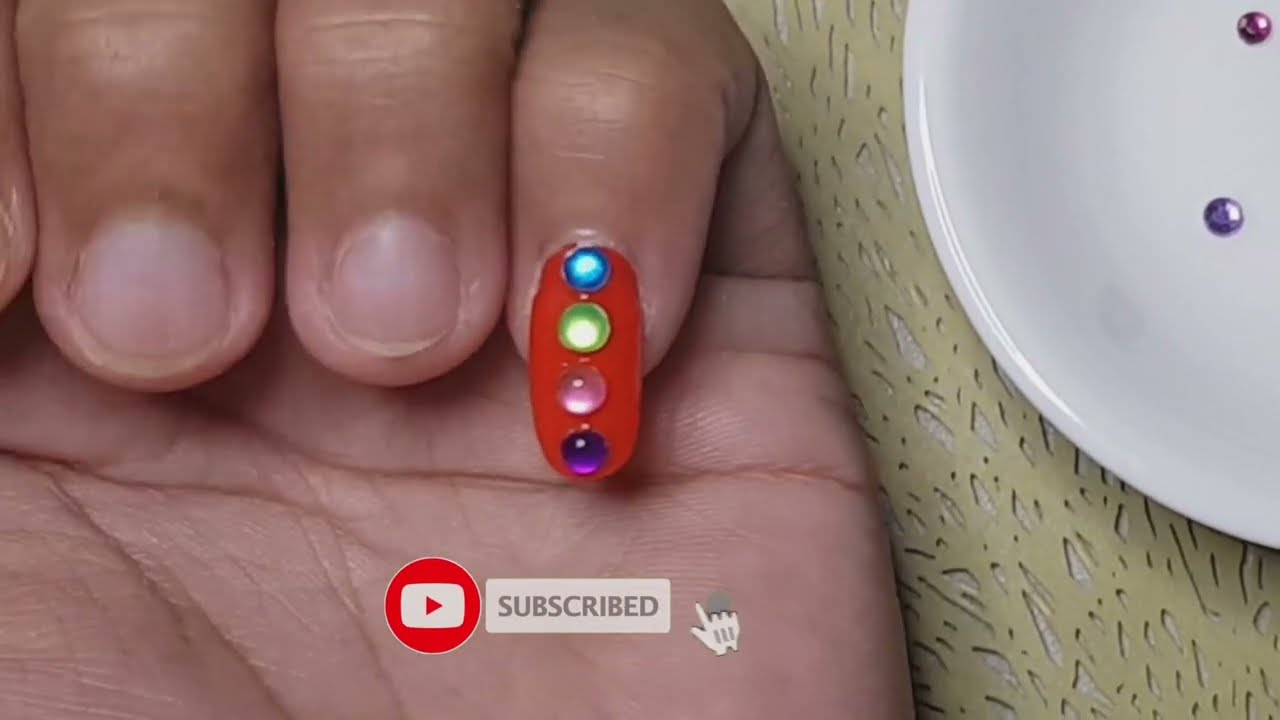The image is a detailed close-up photograph of someone's left hand, palm up, with the fingers curled, showcasing their nails. Prominently, the pinky finger displays a long, red acrylic nail adorned with four plastic jewels arranged in a line: turquoise closest to the nail bed, followed by green, pink, and purple. The middle and ring fingers, in contrast, have short, possibly bitten nails. The hand rests on a surface that appears textured, potentially rubber. To the right of the hand, there is a small dish containing additional plastic gems. At the bottom of the image, there is a YouTube overlay with a play icon, a red circle with a white triangle in the center, and an arrow, along with a bar indicating that the user is subscribed to the channel.